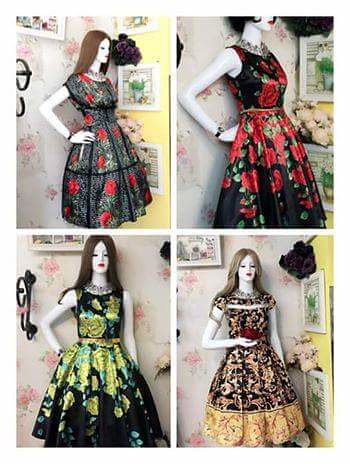This image is a portrait-format compilation consisting of four distinct, equally-sized color photographs of a mannequin against a mix of backgrounds. Each photograph features the same white-skinned mannequin posing with a hand on its hip, dressed in different 1950s-style dresses with fitted bodices and full skirts. 

In the top-left image, the mannequin wears a black dress adorned with black panes and bright red roses with green leaves. The top-right shows a similar black dress featuring cascading large red roses with green leaves. The bottom-left displays a dress with a black background adorned with yellow roses and green leaves, while the bottom-right features a black dress with tan, white, and large bordered patterns. 

The background behind the mannequins consists of a white flowery wallpaper on the left side, evolving into a yellow wall with framed photographs or pictures on the right, including a black wrought iron plant holder contributing to the vintage aesthetic.